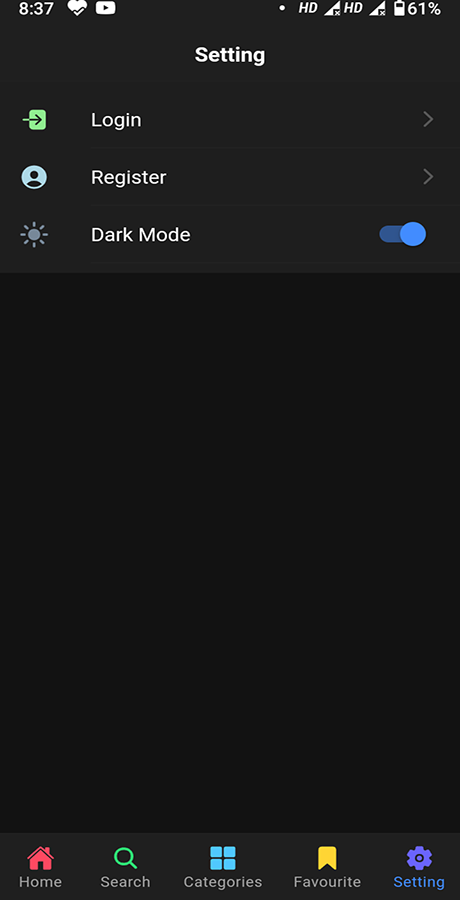Screenshot captured at 8:37 AM displays a YouTube interface with various icons and information. The top section exhibits typical smartphone indicators: signal bars, an HD icon, and a battery level at 61%. Below this, the interface shifts to a larger area with a gray background featuring the word "Satin" prominently displayed in white letters in the center. 

Beneath "Satin," to the left, there is a green square with an arrow and the text "Login," accompanied by a greater-than symbol on the right. Adjacent to this is a light blue circle with a silhouette icon labeled "Register," also with a greater-than symbol. Further down, an icon resembling a light bulb next to "Dark Mode" text indicates a toggle switch that is turned on and highlighted in blue, confirming dark mode activation.

The remainder of the screen is predominantly empty, marked by a large black area. At the very bottom, there is a navigation bar consisting of three icons: a red house symbol labeled "Home," a green magnifying glass for "Search," and four light blue squares grouped under "Categories."